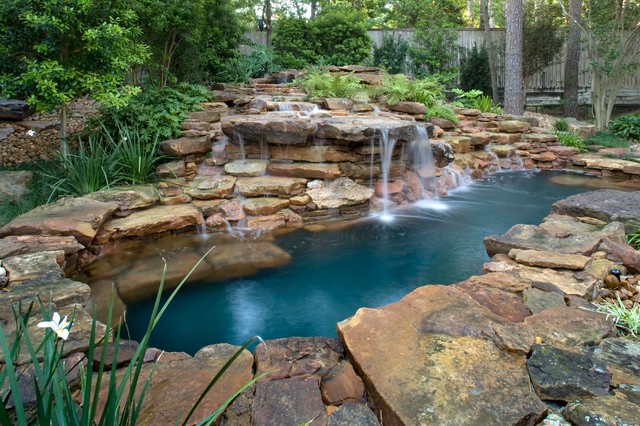The image portrays a tranquil, man-made pond surrounded by a variety of natural elements. The pond is encircled by strategically placed rocks and boulders in shades of brown, beige, black, orangish-brown, yellow, and gray, giving it a natural, yet deliberately constructed appearance. Cascading water flows from a small waterfall at the back of the pond, splashing into the clear, blue water below. The serene setting is enhanced by lush greenery, including full trees with dark and light green leaves. A white fence or wall is visible in the background, adding contrast to the verdant landscape. Off to the left, a delicate white flower with off-white petals adds a touch of elegance. The entire scene is bathed in natural light, creating a calm and soothing ambiance.